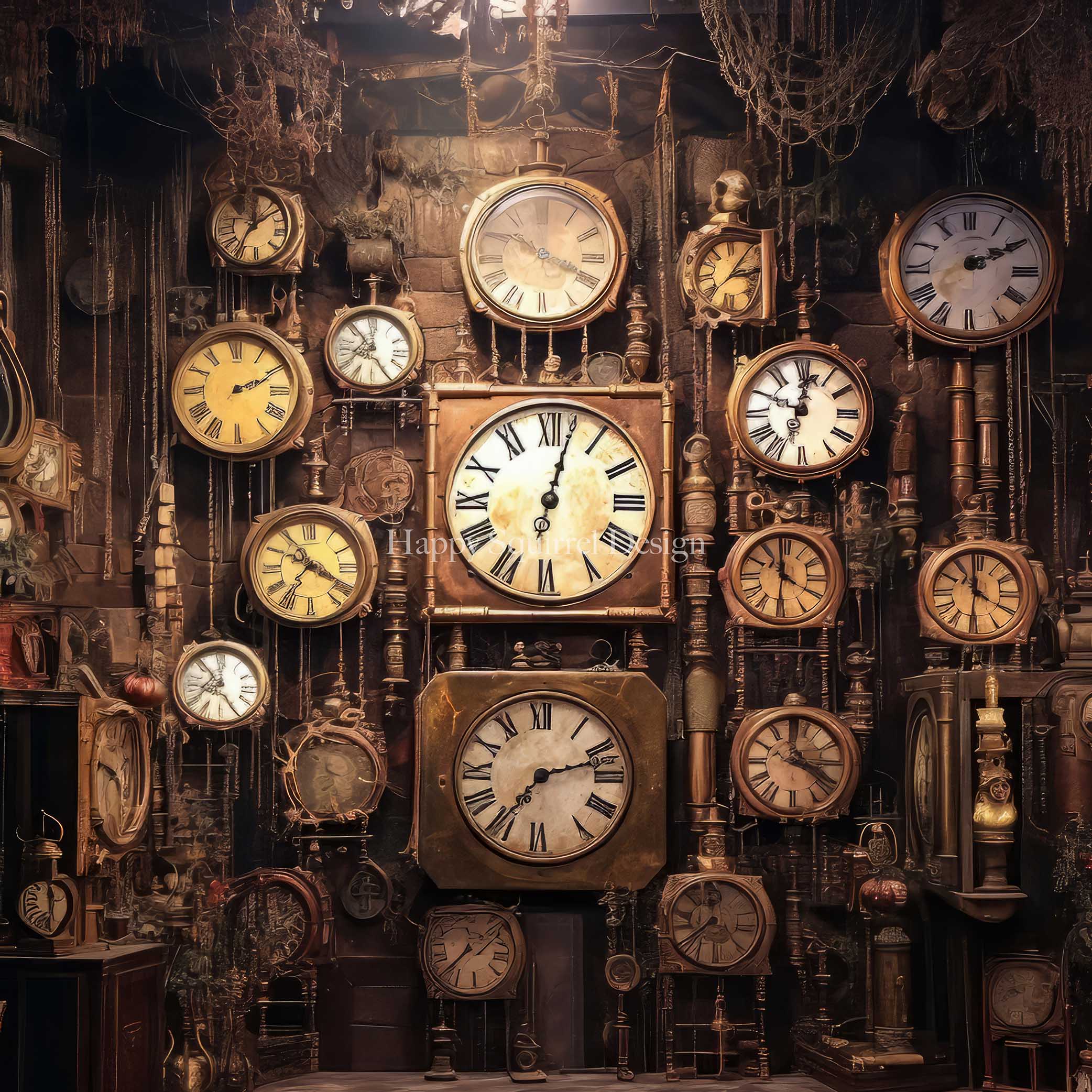This photograph captures a room adorned with a collection of various clocks set against a brownish wall. The clocks, numbering approximately 18 to 20, display a range of styles and sizes, but all feature white or beige faces with Roman numerals and black metal hands. Among these, two larger clocks stand out in the middle, both with circular faces on square golden or brass-colored backgrounds, while another large clock has a simple circular design. The rest of the clocks, reminiscent of grandfather clock faces, are predominantly circular and vary in size. The clocks are arranged in a seemingly mechanical ensemble, all interconnected and partly aged, adding to their vintage aesthetic. The scene is unified by a brownish hue that permeates the image, contrasted by the white or beige faces of the clocks and their intricate, black metal hands. The overall impression is that of an intricate, timeless assembly, blending elements of historical elegance with mechanical precision.